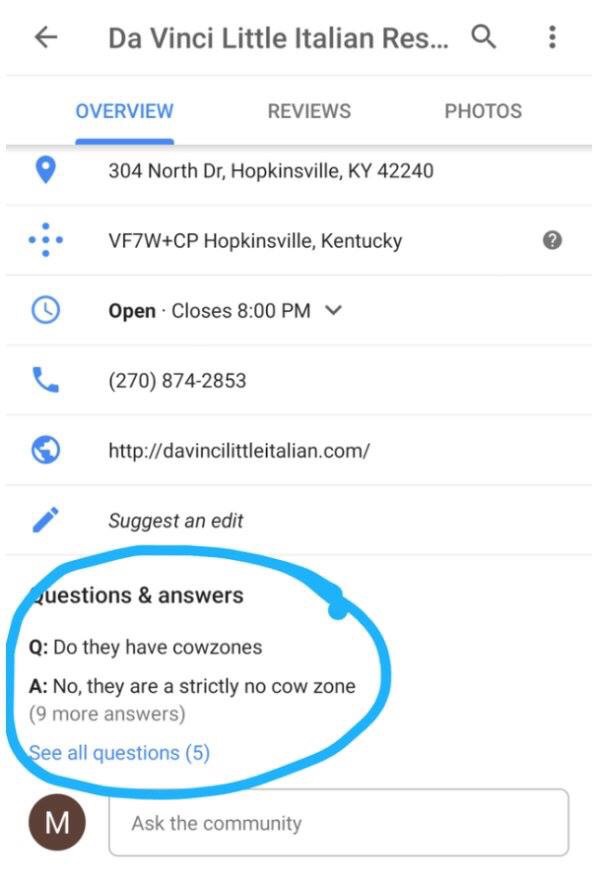A mobile phone screen displaying a search result for "Da Vinci's Little Italian Restaurant" in Hopkinsville, Kentucky. The search overview includes the restaurant's operational hours, indicating it is currently open until 8:00 PM. The result provides the restaurant’s website, "DavinciLittleItalian.com," and lists its contact number. A section featuring reviews from the public and previous customers is visible, alongside a section inviting users to upload photos of the restaurant and its meals. Highlighted in the screenshot is a circled Q&A section specifically addressing whether the restaurant serves calzones, with their strict no-calzone policy emphasized in the response. There are nine additional answers related to the calzone query and a total of five questions posed about the restaurant.